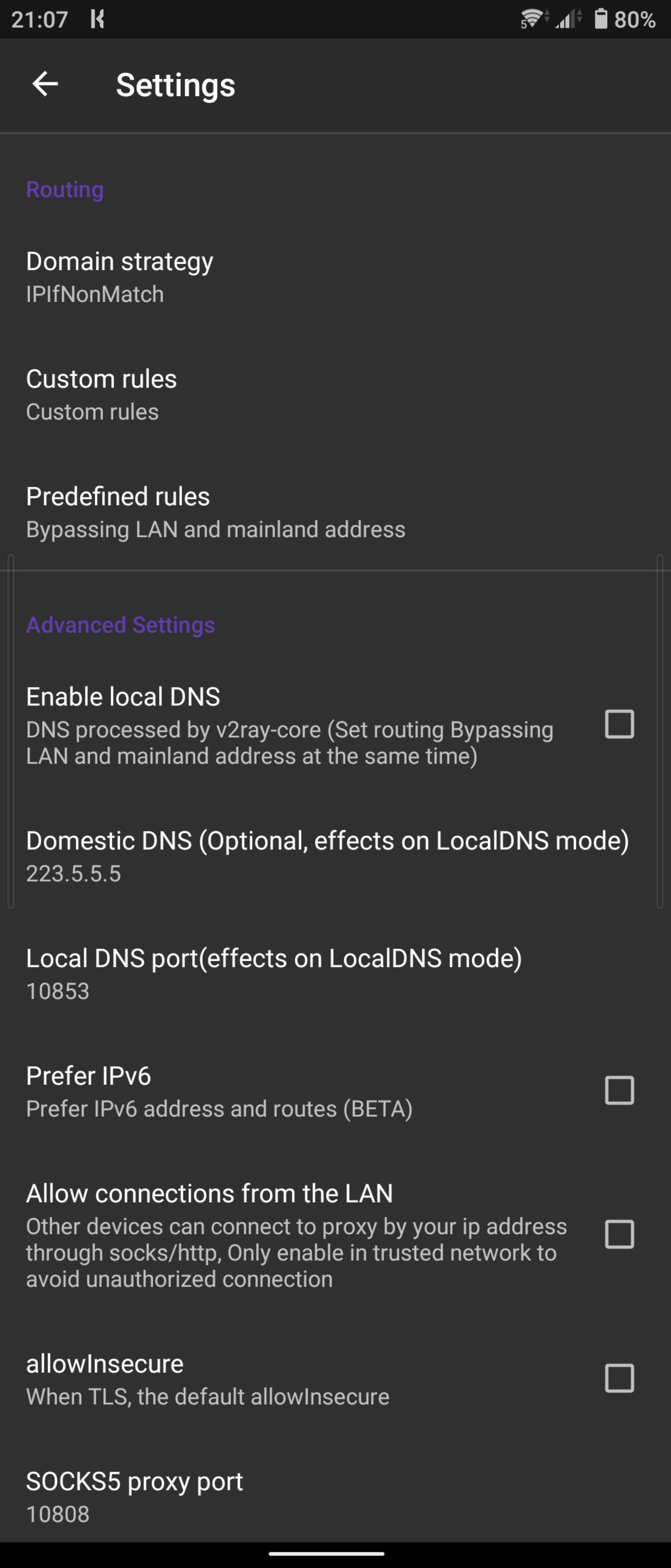The screenshot showcases the settings interface of a device, highlighting various network configurations. In the top left corner, the device's time is displayed as 9:07. On the top right, the status indicators show a full WiFi signal with 4 out of 4 bars, a network signal bar, and a battery level at 80%.

The interface contains multiple settings and options, including:
- "Settings"
- "Routing"
- "Domain Strategy"
- "IP if Non-Match"
- "Custom Rules"
- "Predefined Rules"
- "Bypassing LAN and Mainland Address"
- "Advanced Settings"

Within "Advanced Settings":
- The option "Enable Local DNS" is not selected
- The "Domestic DNS" field is optional and notes the effect on local DNS mode with an entry of "223.5.5.5"
- The "Local DNS Port" is set to "10853"
- "Preferred IP Version 6" is not selected
- "Allow Connections from the LAN" is not selected
- "Allow Insecure" is not selected
- The "SOCKS S5 Proxy Port" is configured to "10808"

This detailed configuration screen provides an in-depth look at the network and proxy settings available on the device.